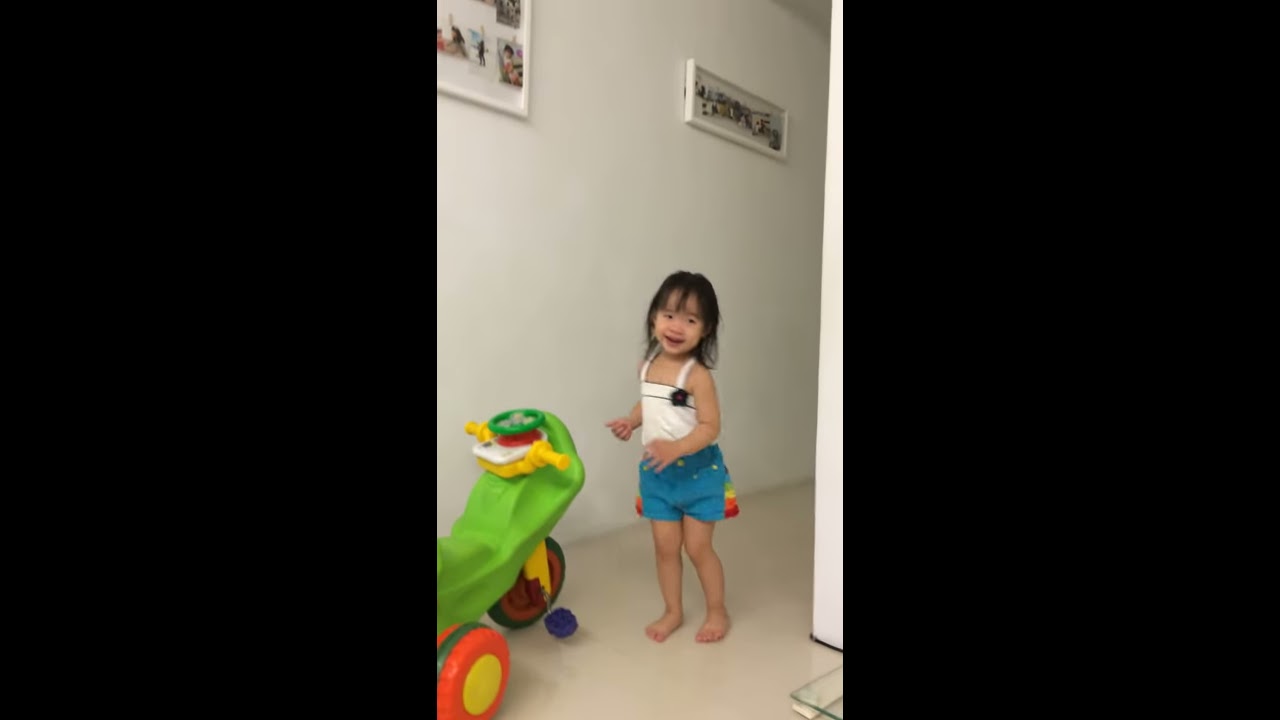This is a detailed portrait-style photograph of a very happy young Asian toddler, around three years old, with shoulder-length black hair and bangs. She is standing barefoot, beaming with a smile, in a room with cream-colored tiles and yellow-painted walls adorned with two collage photo frames. The young girl, who has a light Asian complexion, is dressed in a white tank top with a small flower on the top right, and blue shorts featuring a rainbow pattern on the sides. Nearby, on her left, there's a colorful green tricycle with yellow handlebars and red wheels. Additionally, a little blue ball lies on the ground close to her. The setting appears to be the entrance to a hallway, framed on either side by wide vertical black strips.